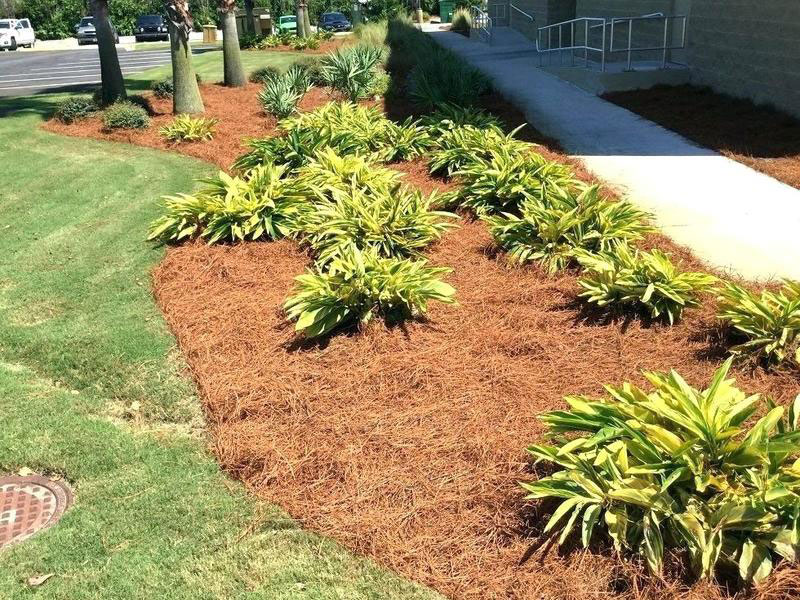The image presents a well-maintained outdoor landscape in front of a building. In the upper right corner, there is a concrete walkway with shiny white railings that lead up to a doorway of the dark gray building, constructed with concrete blocks. Adjacent to the walkway, the landscape features a lush green lawn interspersed with reddish-brown pine straw mulch, where several vibrant green and yellow plants and shrubs grow. Notably, three palm trees with wide brown trunks and dense green foliage rise from the mulch in the upper left corner, behind which a parking lot with clearly marked white lines and a few cars are visible. Additionally, a circular, rust-colored sewer grate can be seen in the lower left corner, set within the verdant grass. The overall scene is framed by continuous bushes and an array of well-tended, tropical-like greenery, creating a visually appealing and orderly environment.